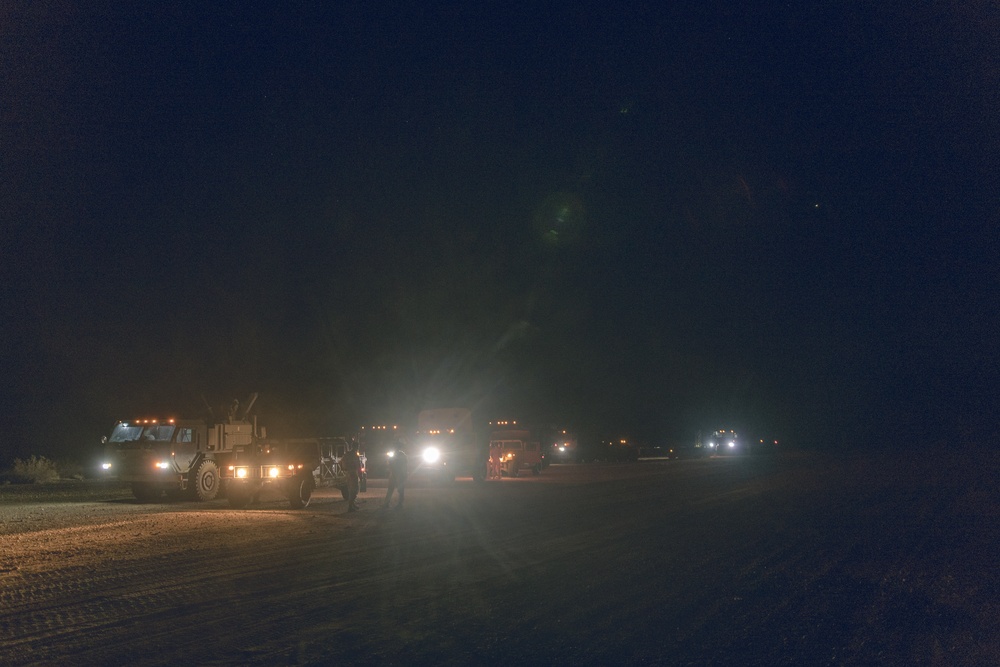In this nighttime photograph, the viewer is taken to a dark, vast desert-like landscape under a pitch-black sky with a single visible star. The bottom third of the scene reveals a wide, sandy dirt road scarred with numerous tire tracks. To the left of the image, a convoy of military vehicles stretches into the distance, their headlights piercing the darkness. At the front of this line, two vehicles drive side by side. The vehicle on the left is a hulking military truck with a high, boxy front and orange lights mounted above, its rear bed shrouded in mystery. Next to it, a squat, square, Hummer-like vehicle reveals its driver sitting behind the engine area. The convoy continues to recede into the horizon, with headlights creating a striking lens flare in the middle of the photo. Sparse human figures can be discerned walking around the vehicles, adding a sense of scale and activity to the otherwise still and expansive nighttime scene.